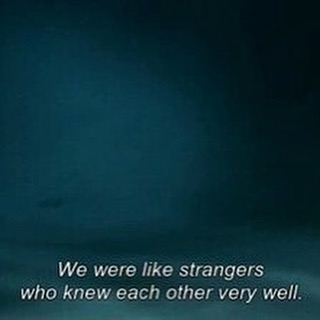The square image has a rich teal background that transitions from an almost pitch-black hue in the top right corner to a lighter teal towards the bottom left. The colors and textures shift, giving an impression of depth and possibly resembling mist or smoke, with some viewers even noticing a faint, misty face. The lower part of the image features white, italicized text in a sans serif font, likely Arial, which reads, “We were like strangers who knew each other very well.” This text is outlined with a black border, giving it a distinct appearance against the varied teal and blue background. The overall atmosphere of the image is reminiscent of an underwater scene or a frame from a documentary, accentuated by its moody, enigmatic presentation.